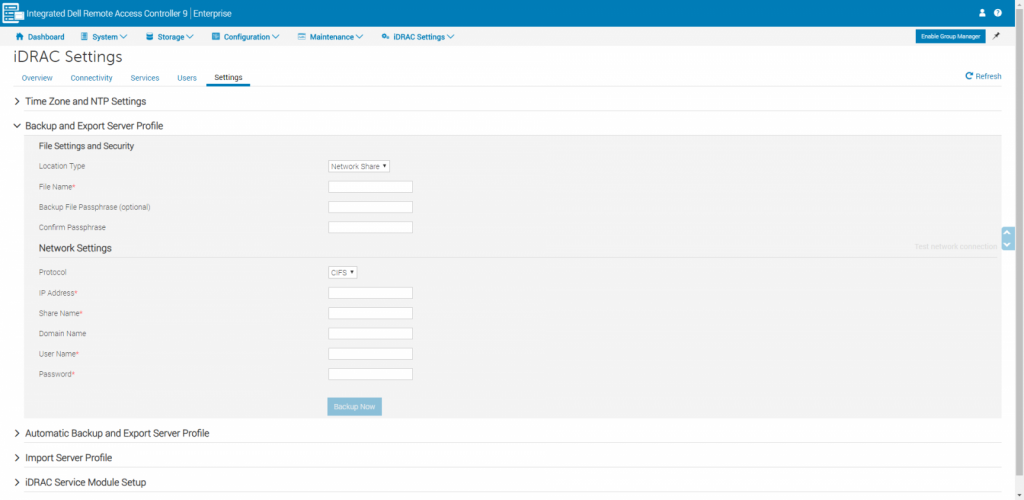Detailed Caption: 

This appears to be an interface for configuring Integrated Dell Remote Access Controller (iDRAC) settings. The page is bordered at the top by a blue band containing the title "Integrated Dell Remote Access Controller Network Line Enterprise." To the far right of this band, there is a white person icon next to a round button. Below the title bar, there are blue text labels accompanied by icons for different sections of the interface including "Dashboard," "System," "Storage," "Configuration," "Maintenance," and "iDRAC Settings."

The main screen is focused on the "iDRAC Settings" section. On the left-hand side, there is a menu listing sub-sections such as "Overview," "Connectivity," "Services," "Users," and "Settings" with "Settings" currently selected. On the right-hand side, under the settings section, there are various configuration options. 

These include fields and settings for "Time Zone and NTP Settings," "Backup and Export," "Server Profile," "File Setting and Security," among others. Specific fields listed here are: "Location Type," "File Name," "Backup File (optional)," "Re-passphrase (optional)," and "Confirm Passphrase." Additionally, it includes "Network Settings" fields such as "Protocol," "IP Address," "Share Name," "Container Name," "Username," and "Password."

Action buttons available on this interface are "Booking," "Backup Now," and options for "Automatic Backup and Export Server Profile," "Import Server Profile," and "iDRAC Self-Service Modular Setup." Despite the enlargement of the image to 177%, some sections, especially those encapsulated in a blue box on the right, remain blurred and unreadable.